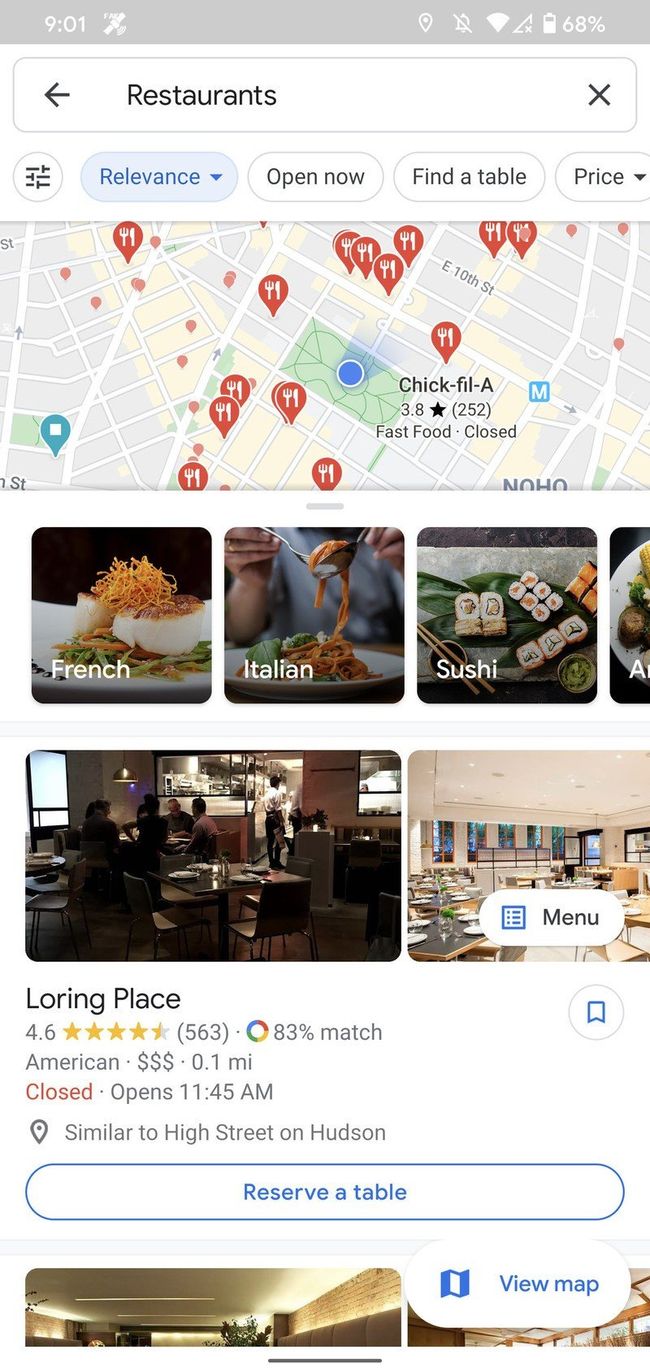The image displays a smartphone screen with a detailed restaurant search interface. At the top, there's a gray status bar featuring the time "9:01" in white lettering on the left. On the right side of the bar, there is a notifications icon with a diagonal line through it, a Wi-Fi symbol, and cell signal bars marked with an "X" at the bottom right corner. The battery level is shown at 68%.

Below the status bar, on the left, there's a black left arrow icon labeled "Restaurants," followed by a close (X) icon. Under these, the interface lists filters such as "Relevance," "Open Now," "Find Table," "Price," with a map filled with numerous red markers representing different restaurant locations.

Further down, the screen presents three photograph sections categorized under "French," "Italian," and "Sushi." Below this, a restaurant listing for "Loring Place" is displayed prominently with accompanying details: it has a rating of 4.6 stars from 563 reviews, shows an 83% match, is categorized as American cuisine, indicated by three dollar signs, located 0.1 miles away, currently closed, and opens at 11:45 a.m. There is a comparison to a similar restaurant, "High Street on Hudson," and an option to "Reserve a Table" through a white button outlined in blue with blue text.

Beneath the Loring Place listing, two additional photos are partially visible, cut off by a white button with blue text labeled "View Map." The red markers on the displayed map indicate various restaurant locations.